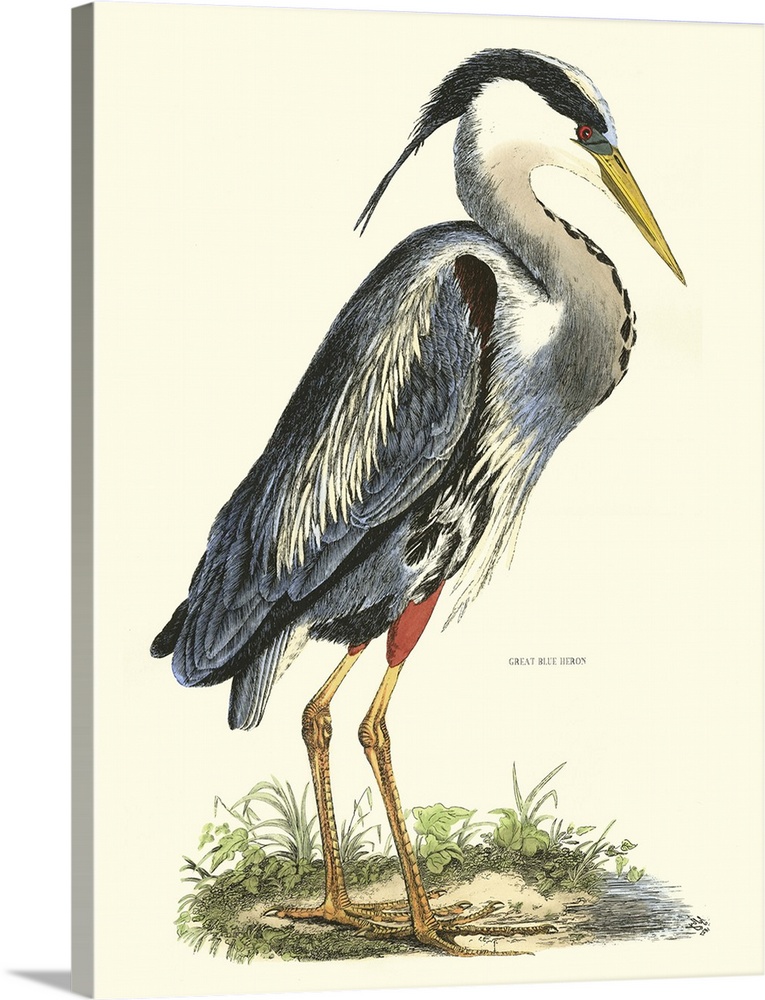The image is a detailed illustration of a majestic great blue heron, set against a light yellow, cream-colored background. The bird stands on impressively long, yellow legs that are straight and slightly spread out at the claws. The top sections of the legs feature dark orange hues. The heron's body showcases a mix of dark black and dark blue feathers interspersed with patches of white plumage. Its long neck, light gray in color, extends prominently to the right before curving gracefully back to the left and upwards, with the head directed down towards the right side. The heron's head is adorned with a striking black crest, and it has a vivid red eye and a yellow beak. The bird's tail feathers trail downwards towards the bottom left of the image. Surrounding the heron is a ground surface dotted with both green and dead black vegetation, adding to the natural setting. Beneath the drawing, there is a signature that begins with "Great" but ultimately the rest of it is too small to decipher. The combination of detailed feather coloring and natural elements in the background make this illustration both vibrant and captivating.